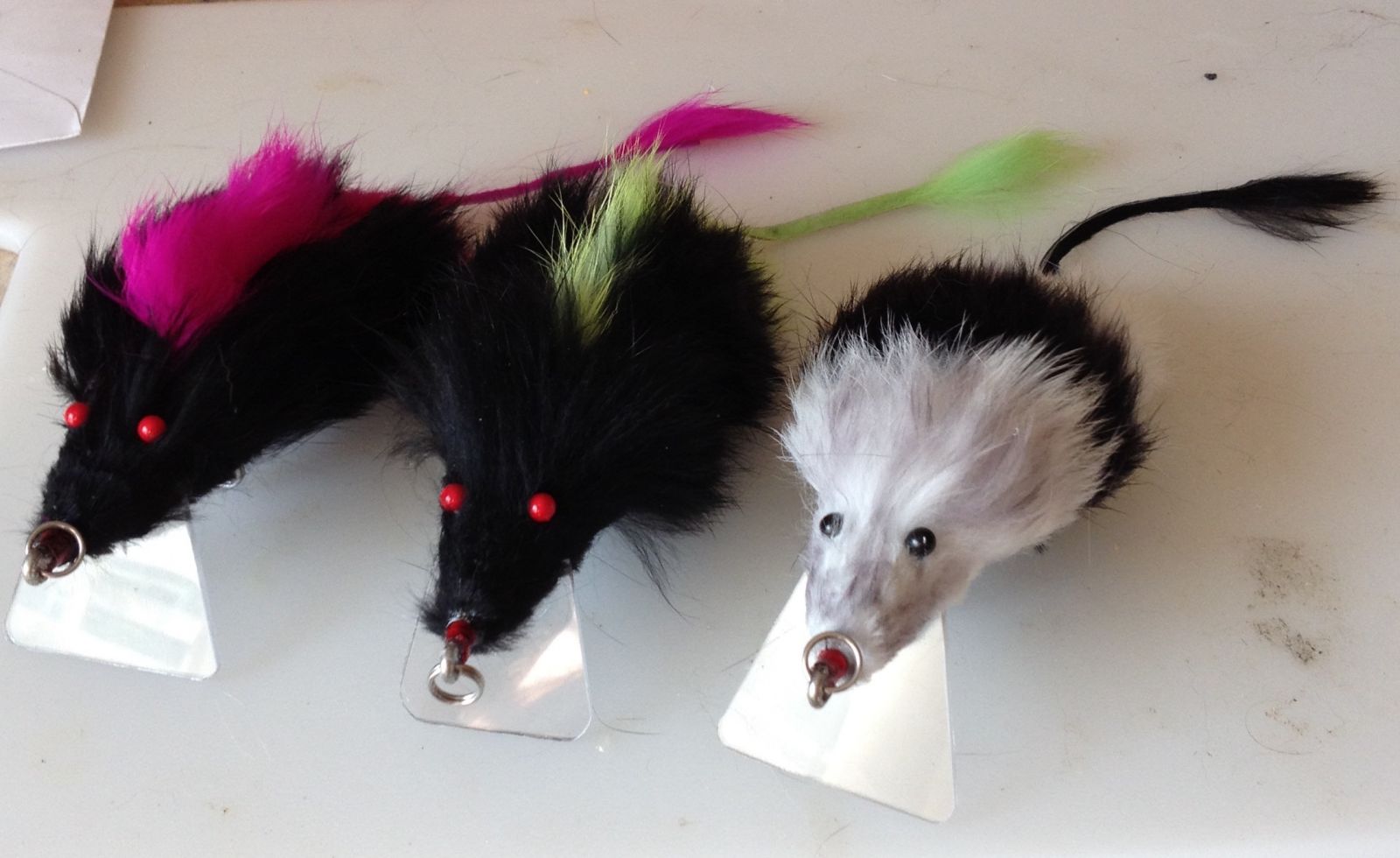The image depicts three small stuffed animal rats arranged horizontally on what appears to be a marbled white countertop. From left to right, the first two rats are black with vivid red eyes, each adorned with a distinctively colored Mohawk and corresponding tails—one with bright pink and the other with vibrant green. The third rat is the most unique, sporting a white face and front, with its fur transitioning to black towards the back, ending in a black tail. All three rats have beaded eyes, long pointed snouts, and a silver metal ring hanging from their noses. They appear to be supported by small, triangular stands beneath their noses and mouths. The surface is marbled with black smudges, and a noticeable dark smudge is situated on the right side of the desk.